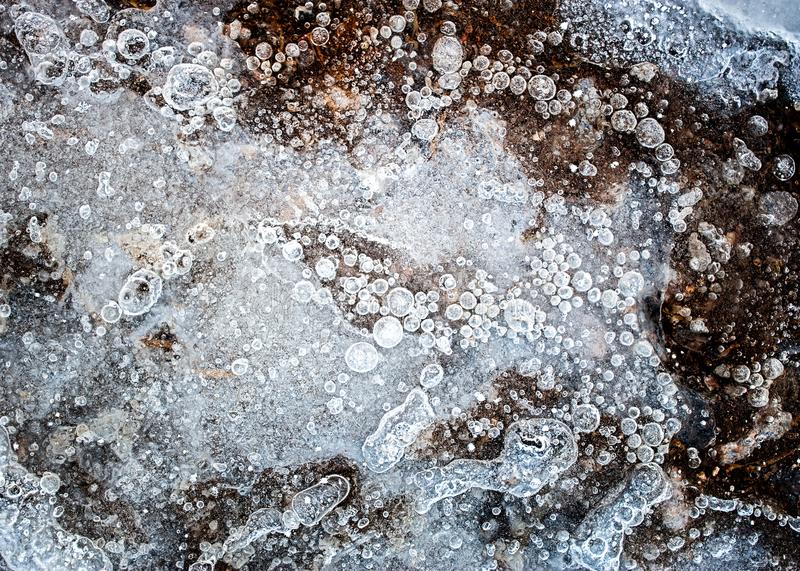This highly detailed color photograph captures an abstract and intricate frozen landscape. It reveals an extensive field of bubbles, strikingly solidified in a variety of shapes and sizes. The image evokes the appearance of a frozen ground near a river or lake, interspersed with hundreds of microscopic-sized, white, yellow, and orange orbs, with subtle tinges of blue. The background underneath the frozen bubbles features a rusty brown hue, creating a stark contrast. The bubbles, which are uniformly distributed across the surface, bear a resemblance to the view one might expect under a microscope, presenting an almost biological appearance, like frozen microbes. The composition lacks a clear sense of scale, adding to the enigmatic quality, and on the right-hand side and lower left, larger brown areas emerge, hinting at the ground beneath water splashes halted in time. The photograph, with its combination of earthy tones and frosted formations, conjures images of a topographical map or a snapshot of a natural phenomenon, captured in an up-close, almost surreal perspective.